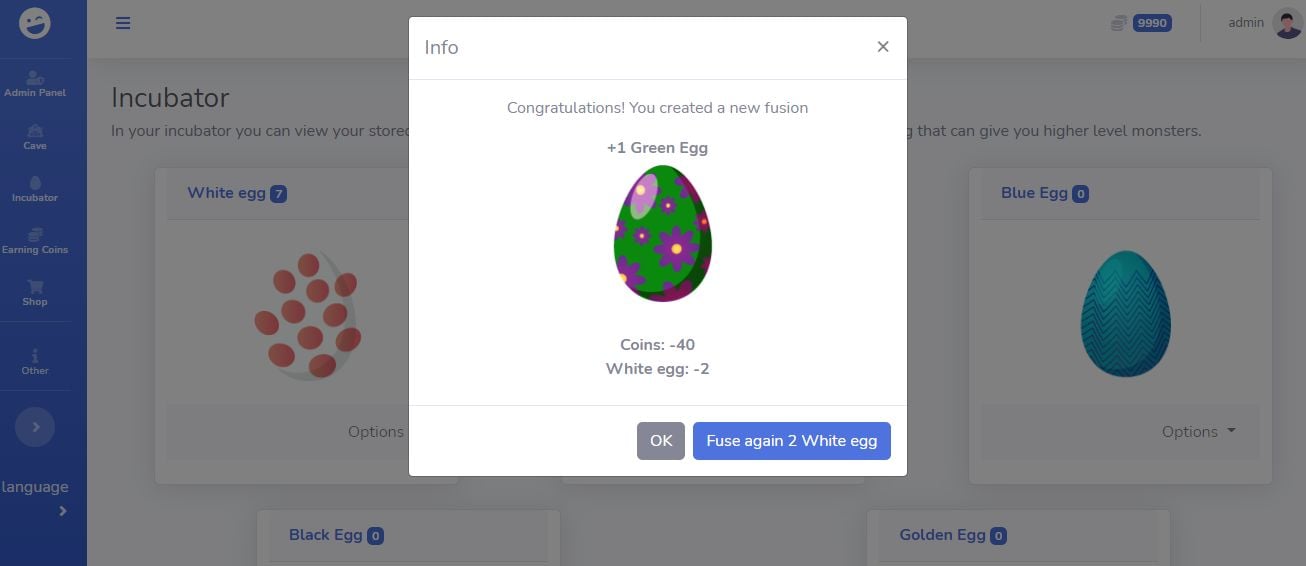This image is a detailed screenshot from a game, featuring both the gameplay interface and an informational overlay. The background of the image is predominantly white, with a blurred blue banner on the side. 

At the top of the overlay, positioned as a square, there is light gray text that reads "Info". Below this, a thin gray line separates the header from the rest of the content. The next text line, in bold, states "Congratulations!" followed by "You created a new fusion." This is further highlighted by details underneath stating "+1 Green Egg," accompanied by an image of a green egg adorned with purple flowers that have yellow centers.

Further below, the text notes "Coins: -40" and "White Egg: -2" to indicate the resources spent. Another thin gray line separates these details from two interactive buttons at the bottom. On the left is a small gray square button labeled "Okay" in white letters. On the right is a larger rectangular button featuring a blue background and white text that reads "Fuse again (2 White Eggs)." There is also an 'X' in one corner to close the overlay.

In the blurred background, the word "Incubator" is visible, with the phrase "In your incubator, you can view your store" written underneath. There are highlighted sections with blue text including "White Egg," showing an image of a white egg with orange circles, and another section labeled "Blue Egg," depicting a tealish blue egg within a square.